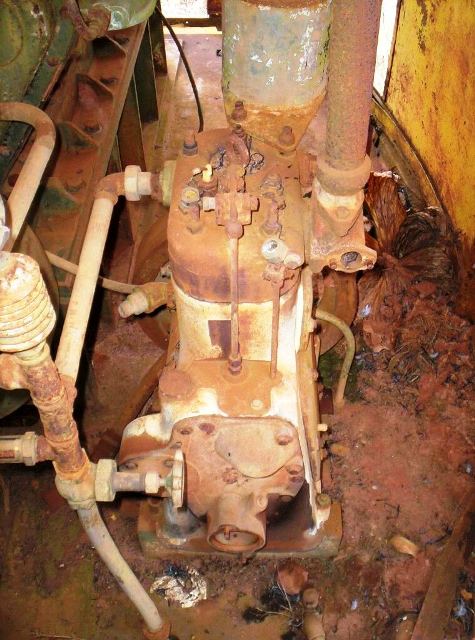The image depicts a severely rusted, industrial-like mechanical apparatus, possibly an HVAC system or pump with extensive corrosion covering nearly all surfaces. The machinery seems to have originally been white, evidenced by faint speckles of paint peeking through the rust. The apparatus is centrally located, featuring multiple pipes – including a prominent circular pipe emerging from the top – and a horizontally-aligned white pipe that bends forward and then upward. To the left, additional metal components like valves and handles are visible, while a green metal object appears to be connected to the main system. The ground beneath the machinery is muddy and grime-filled, littered with rust debris and possibly organic material in advanced decay, contributing to an overall unsanitary and unsafe environment, lacking proper containment and maintenance.